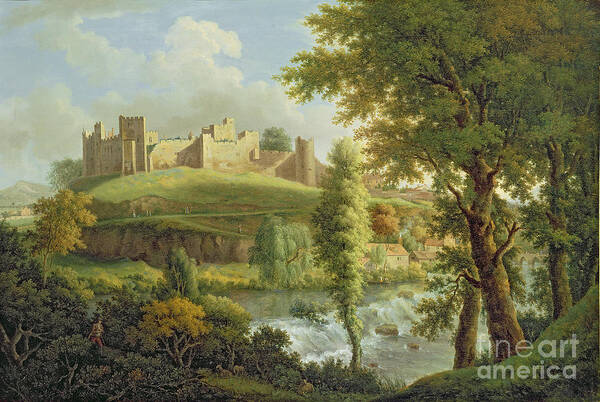The painting depicts a scenic outdoor setting dominated by a majestic castle perched atop a cliff overlooking a body of water. Behind the castle, a range of mountains rises, framed by a backdrop of green trees and fluffy clouds against a serene blue sky. The castle itself features prominent towers and a turret on the right side, with what appears to be a sloping wall, possibly a staircase, leading to the turret. 

In the foreground, dense greenery envelops the scene. On the right-hand side, three or four massive trees stand in a row, opposite a spindly tree at the center and various bushes along the left side. Below the castle's cliff, the water rushes, producing foam where waves crash, and there is a noticeable rock amidst the flowing water. The bottom right of the image is marked with the text "Fine Art America," signifying the artwork's source.